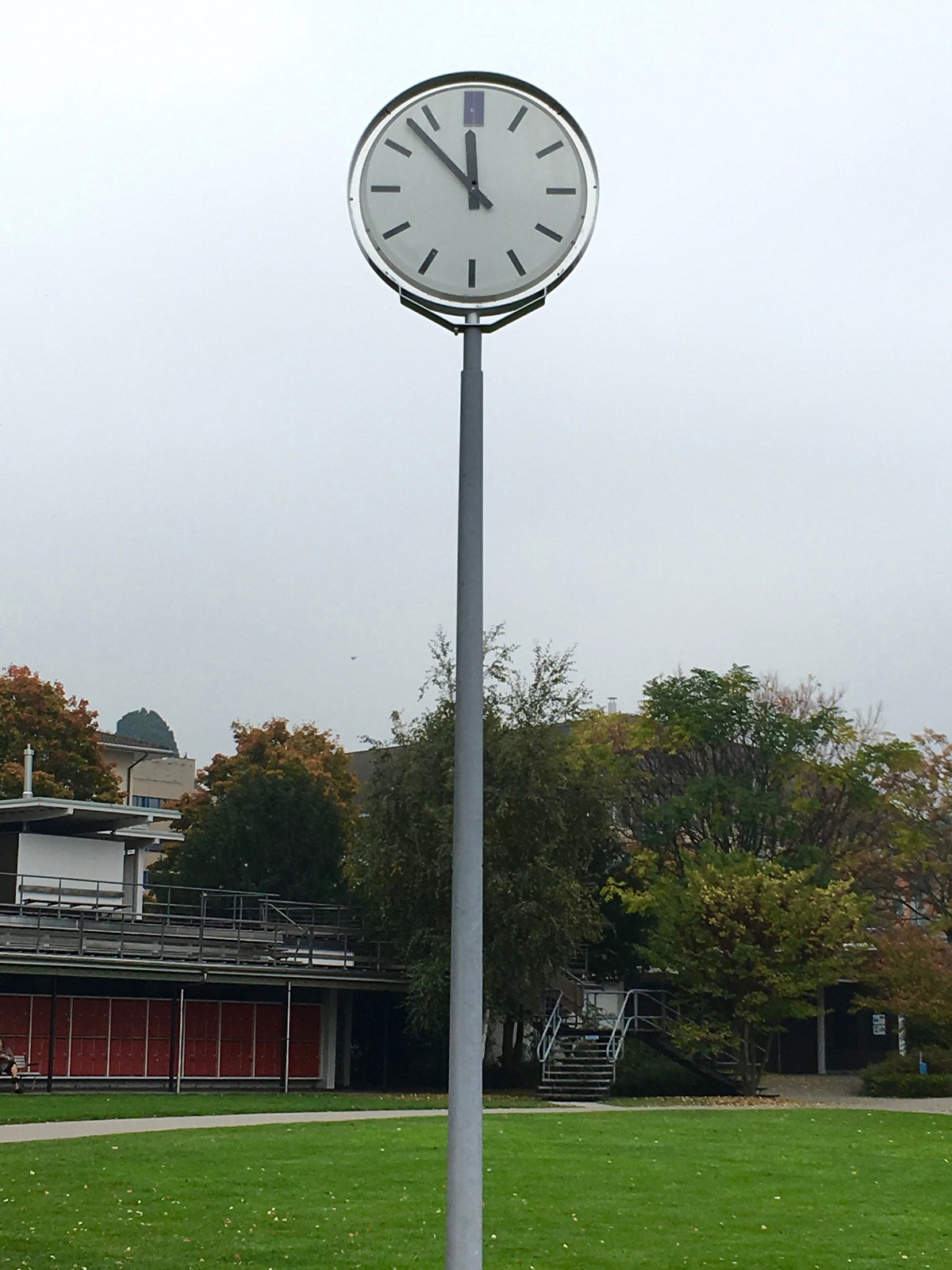In this outdoor photograph, a tall, slender gray pole supports a silver-framed clock with a white face. The clock, which lacks traditional numbers, instead features minimalist slashes to mark the hours. The time displayed is close to noon. Beneath the clock, a well-maintained, lush green field stretches out, emphasizing meticulous care. In the distance, an array of trees lines the horizon, adding to the scenic beauty. A building, likely a school, is visible, complete with metal stands and a staircase. To the right of this building, an open courtyard is marked by distinctive white posts.